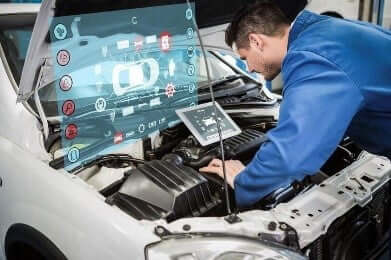The image is a horizontally aligned rectangular photograph of a mechanic, dressed in a blue denim long-sleeve shirt, working on the engine of a white sedan with the hood up. The man, sporting short brown hair that is slightly longer on top, is leaning over the black engine compartment and focusing intently on a small touchscreen device attached to the car's interior, resembling an iPad with a silver rim, displaying a black-and-white image of a car. Above this touchscreen, there is a large computer-generated holographic display featuring a top-down view of a car surrounded by various icons and buttons, with a blue-green, semi-transparent background that evokes a sense of augmented reality. The rod supporting the hood is visible, jutting up vertically on the left side. Below the hood, elements like the wheel well and part of the tire are visible, emphasizing the mechanical focus of the scene.